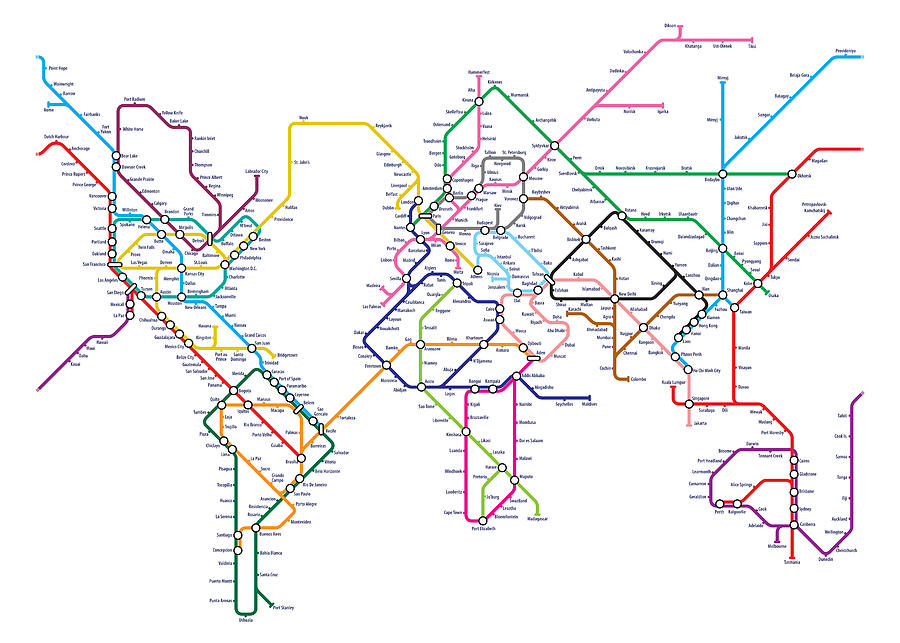The image is a detailed map of a transit system, likely depicting either a subway or bus line network in a city. The map features a complex array of squiggly lines in various colors, including blue, green, yellow, pink, orange, purple, red, and different shades of these hues. Each line represents a different route within the network, and they converge at numerous intersections marked by white circles. These circles indicate stops, with black text next to them naming each stop, although the text is too small to be legible.

In the upper right corner, a blue line extends leftwards before sharply descending towards the left, ending at a white circle. From this point, a green line runs horizontally from left to right, intersecting with an orange line that ascends slightly to the right before extending straight to the right edge of the map. The center of the map is densely packed with intersecting lines and stops, suggesting it is a major hub within the transit system. The left side of the map is also heavily populated with numerous lines and stops, while the right side has fewer stops overall. The background of the map is plain white, providing clear contrast to the vibrant, multi-colored network of transit routes.